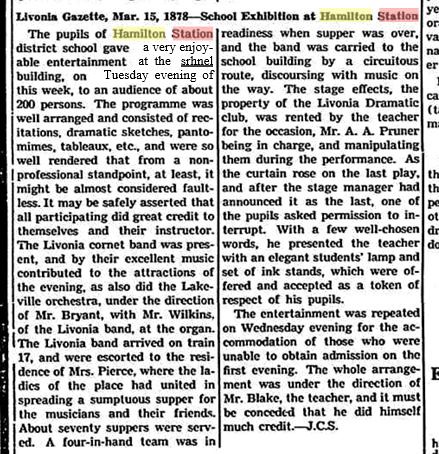This image captures a zoomed-in portion of a newspaper, specifically the "Livonia Gazette" dated March 15, 1878, with a headline about a "School Exhibition at Hamilton Station". The article is divided into two paragraphs with a thin vertical black stripe separating them. "Hamilton" and "Station" are highlighted in yellow and red respectively throughout the text. The left side starts with "The Pupils of Hamilton Station," also using the same highlight scheme for "Hamilton" and "Station". The pupils from the Hamilton Station District School hosted a delightful entertainment at the Schnell Building on Tuesday evening for an audience of about 200 people. The program featured recitations, dramatic sketches, pantomimes, and tableaus, all well-executed to a highly commendable standard. Additional highlights include the Livonia Cornet Band and the Lakeville Orchestra, directed by Mr. Bryant with Mrs. Wilkins at the organ, both contributing significantly to the evening’s success. Following their arrival by train, the band was treated to a lavish supper arranged by local ladies at Mrs. Pierce's residence. The band then performed en route to the school building. The Livonia Dramatic Club provided stage effects managed by Mr. A.A. Pruner. The performance concluded with a pupil presenting their teacher with a student's lamp and ink stands as tokens of respect. Due to high demand, the event was repeated on Wednesday evening. The entire event was skillfully organized under the direction of Mr. Plake, the teacher.